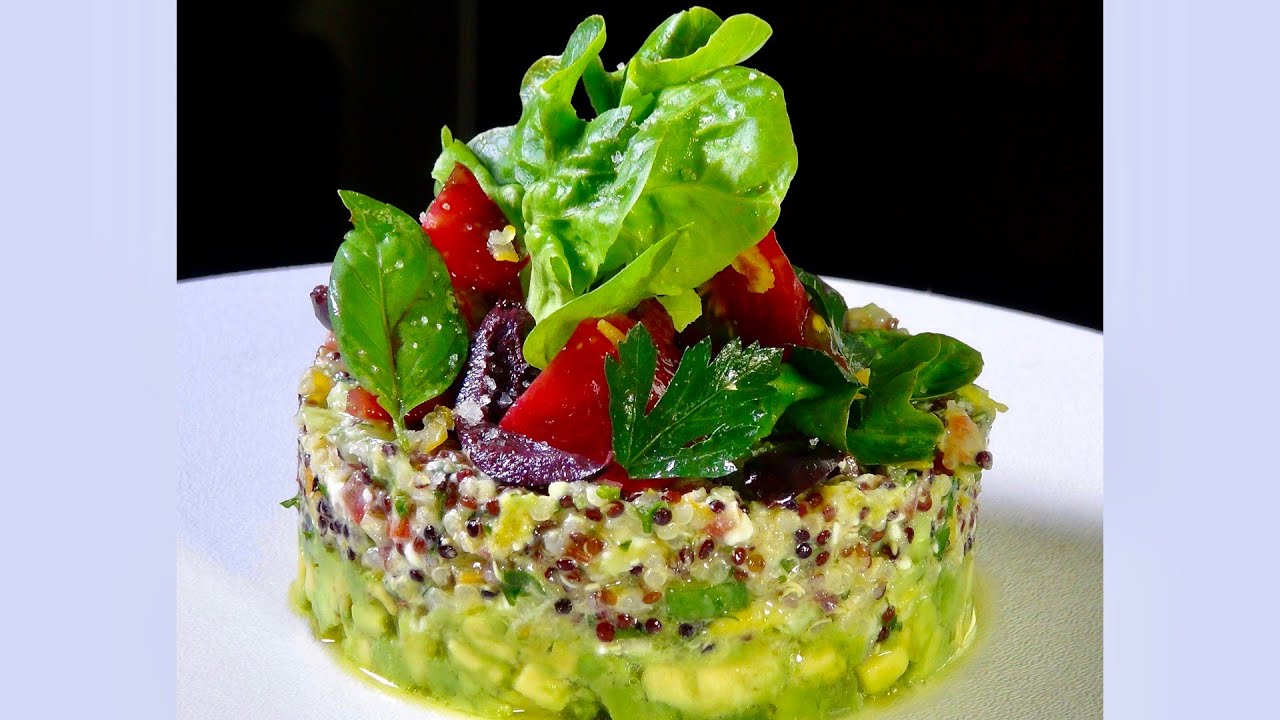This detailed close-up photo captures a vibrant and fresh vegetarian appetizer set on a white plate, dramatically contrasted against a black background, with light blue vertical borders on the left and right sides of the image. The dish resembles a tricolored quinoa turret, possibly shaped using a metal ring, and is layered with a variety of colorful ingredients. The bottom layer consists of mashed avocado, creating a rich green base. This is topped with a mix of vivid ingredients including light green, dark green, purple, yellow, and red colors. Among these, diced red pieces that appear to be tomatoes or red peppers, as well as purple elements that might be beetroots, are easily identifiable. The top is adorned with green leafy components, described as appearing somewhat slimy and possibly resembling lettuce. The overall presentation is visually striking, with the myriad of colors—from greens to reds to purples—creating a visually appealing and mouthwatering appearance, making the dish look incredibly fresh and appetizing.